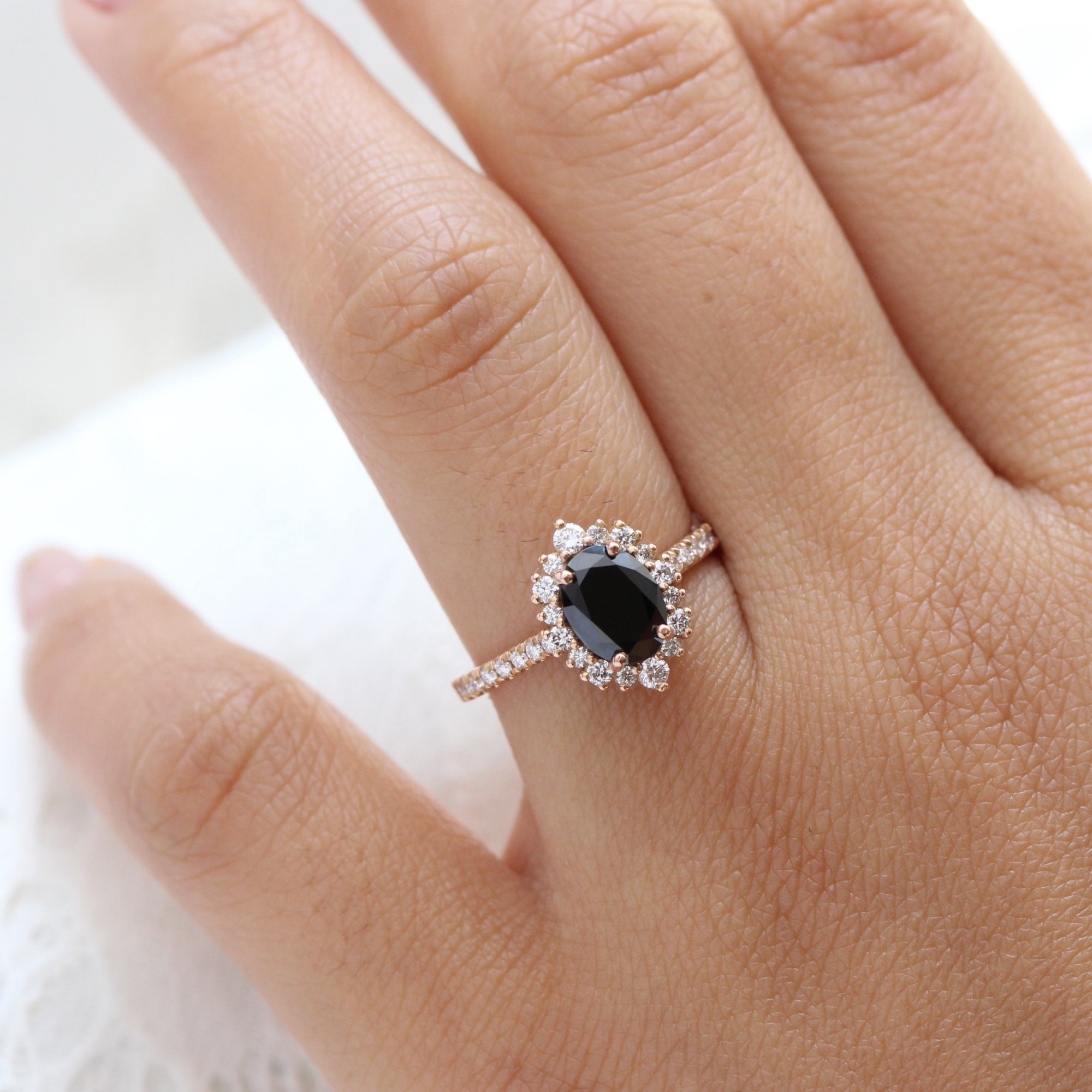The image is a close-up of a light-skinned, possibly Caucasian female hand, prominently displaying an elegant and detailed ring on the ring finger. The ring, likely made of gold, features a large, dark blue or black gemstone at its center, encircled by approximately 15 small diamonds. The band of the ring is also encrusted with several dozen tiny diamonds, adding to its luxurious appearance. The fingernails appear to be painted in a pale pink color. The hand, clearly showing individual wrinkles, rests on a white, soft material, possibly a cloth, that serves as the background for the photograph. The ring's intricate design and the way it's positioned suggest it could be a wedding or engagement ring.